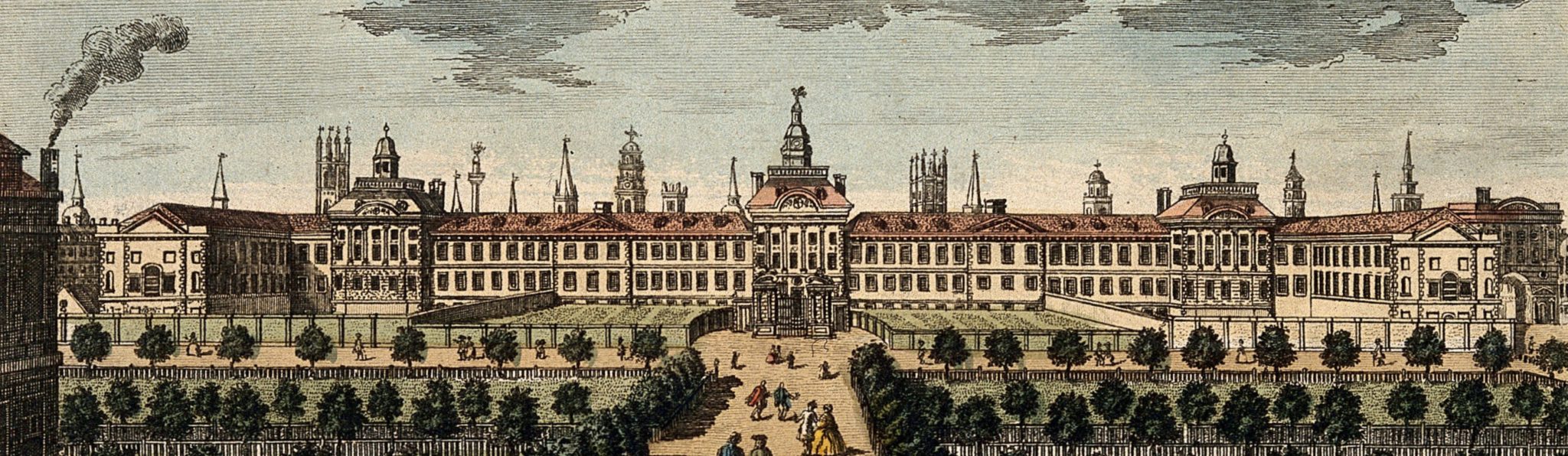The image is a detailed, colored artwork likely depicting a large architectural complex, possibly a palace or historical government building, with a vast number of windows and multiple stories. Structured in a long horizontal rectangle, the building stretches across from the left to the right of the image, characterized by its light tan walls and reddish-orange roof. Prominent towers with crosses are spread across the building, including two smaller ones on the ends and a larger one in the center.

In the foreground, a central path runs from the bottom middle of the image up to a gate, leading to the main entrance of the complex. Flanking this path, lush green lawns are adorned with a variety of trees, which seem to continue into a central courtyard. The courtyard is bordered by green walls and gardens filled with shrubs.

People can be seen walking along the paths, adding life to the scene. To the far left of the image, a smokestack not part of the main building emits a trail of smoke, drifting to the right. The sky above is painted in shades of light blue and gray, with darker, ominous clouds gathering at the very top, adding a muted, almost nostalgic tone to the whole scene. مش